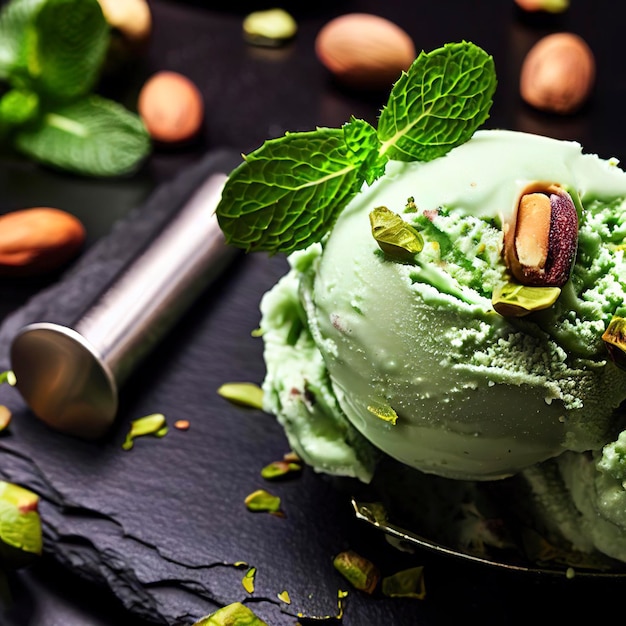This is a detailed close-up shot of a delectable scoop of green pistachio ice cream, adorned with a fresh mint leaf and what appears to be chunks of pistachios or other nuts. The scoop is presented on a dark, stone-like base which might resemble volcanic rock or chocolate. The base is reflective, adding a touch of elegance to the presentation. Complementing this setup is a silver-colored tool with a rounded end, possibly used for serving or garnishing. Scattered around the base and subtly visible in the background are additional nuts and mint leaves, enhancing the intricate and fancy display of this dessert. A piece of chocolate candy with caramel inside also sits atop the scoop, adding further contrast and allure to the composition.